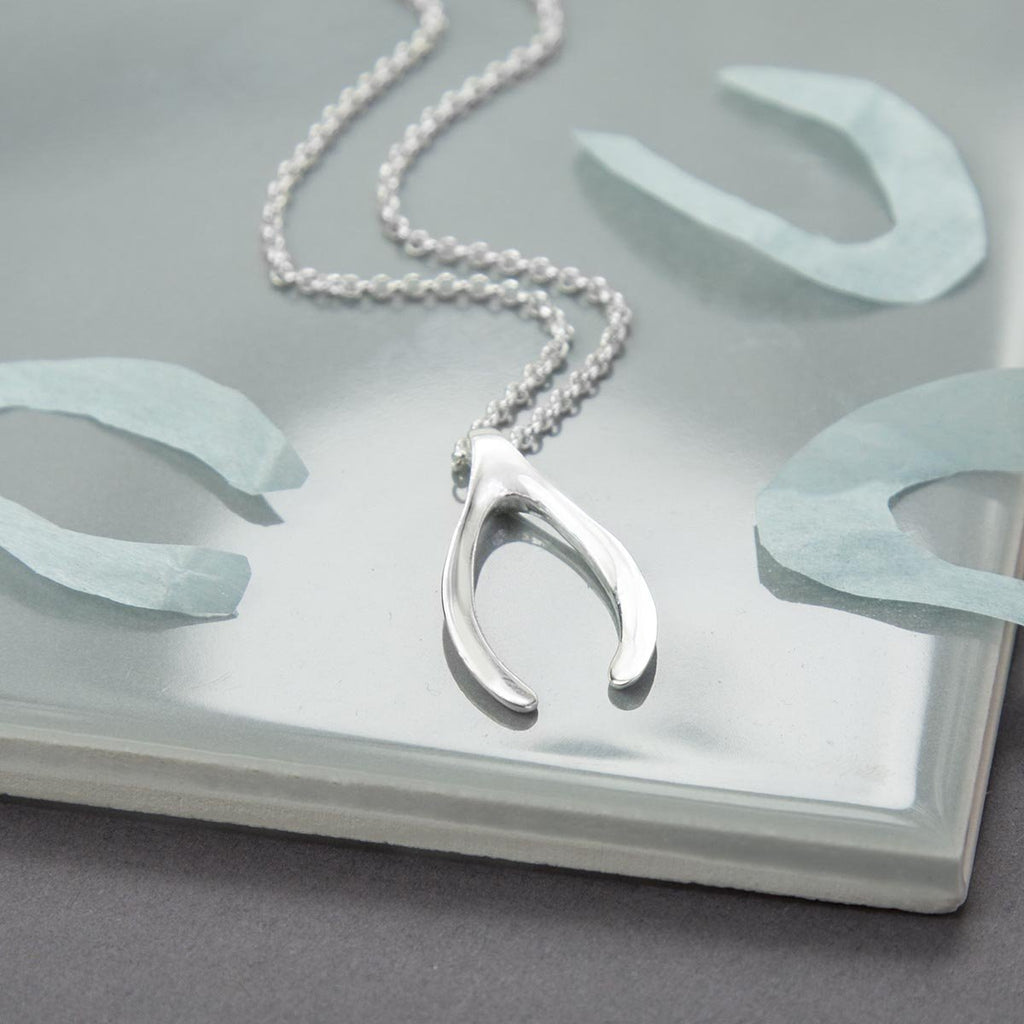This detailed image presents a close-up, square-oriented, 45-degree top-down shot of a reflective, light grey surface. The main subject is a delicate silver wishbone pendant, part of a silver chain necklace, lying against the reflective surface. Surrounding the pendant are three light blue, U-shaped paper cutouts — one fully within the frame on the left, and two partially captured on the right. The reflective quality of the surface suggests it could be glass or a shiny, plastic-like material, showing a reflection of the wishbone pendant. The chain is arranged with a slight spread, emphasizing the elegant wishbone at the bottom center. This careful arrangement on a neutral background highlights the contrast between the silver pendant and the blue paper cutouts, all framed by a darker grey outer surface, creating a visually appealing composition.